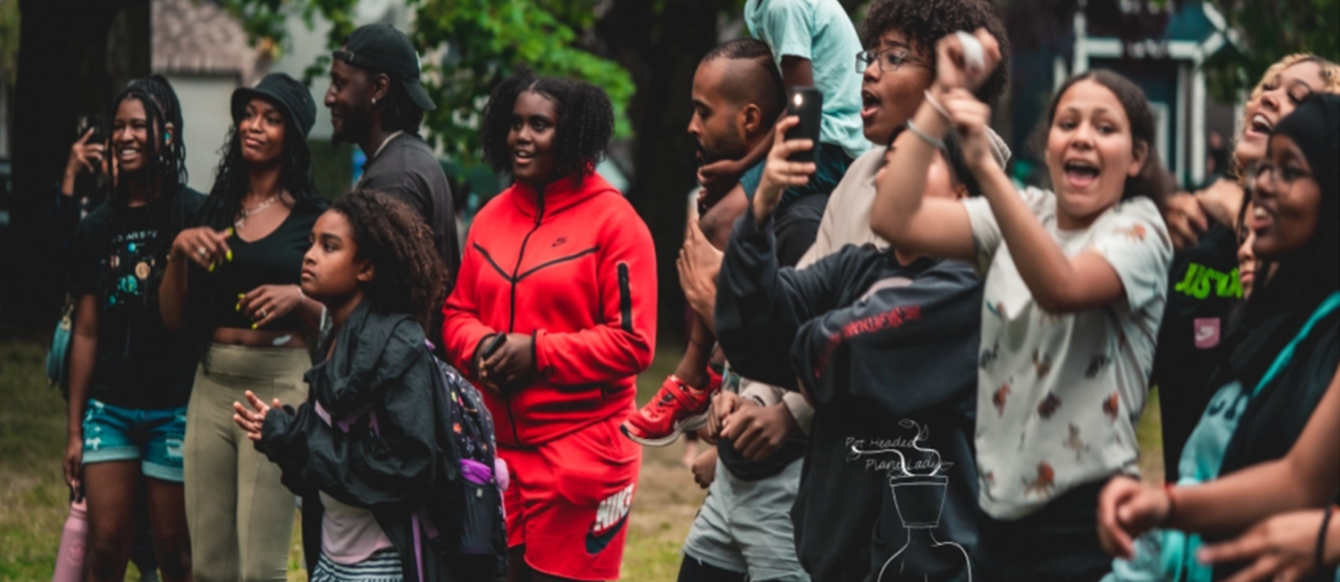In this outdoor scene, a diverse crowd of around thirteen people, including a mix of Black and Latino individuals, are gathered on a grassy area. Two distinct buildings form the background: one is stone-colored with a brown roof, and the other is a brown brick building featuring a white front porch. A lush green tree with abundant foliage stands near the stone-colored building. The crowd, comprising both boys and girls, mostly young, are uniformly focused in one direction, many with cell phones raised to take photos or videos. Interestingly, one boy sits on an adult's shoulders, likely his father, to get a better view. The atmosphere is vibrant and filled with excitement; people are smiling, laughing, and cheering, with expressions ranging from joy to awe. Attires vary from jackets and long sleeves to shorts and short sleeves, suggesting a mix of personal comfort choices. The presence of a tracksuit and a hoodie further highlights the casual, everyday clothing of the group. Despite their legs being cropped out of the frame, the overall scene exudes a lively outdoor activity, possibly a sporting event or a street performance, captivating the entire crowd.